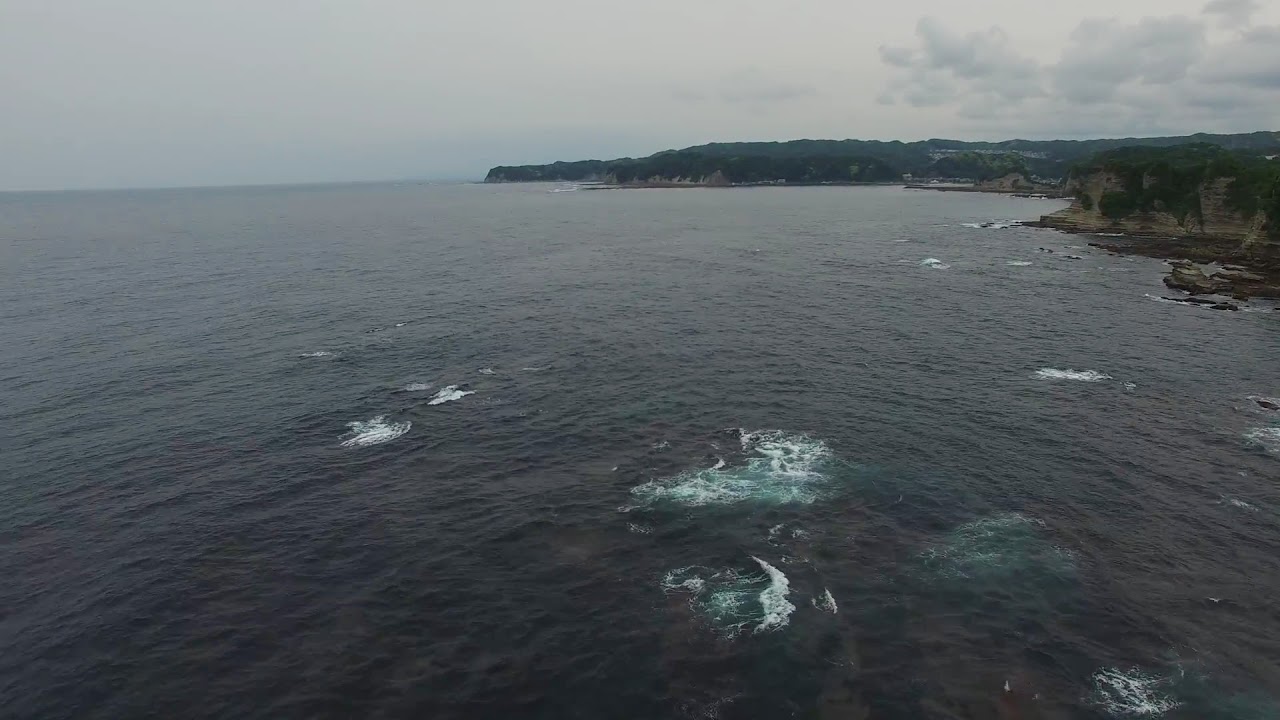The image portrays a vast, dark body of water extending across the lower two-thirds of the scene, exhibiting a spectrum of colors from deep blue to blue-green in areas of disturbance where foamy, white-capped waves ripple towards the foreground. Dominating the right-hand side is a rugged, dark gray cliffside that slopes gradually as it extends into the distance, its steep, tan rock walls adorned with dense green foliage and scattered shrubbery. A tiny island floats near the cliff, slightly above the center-right edge. The sky overhead is heavily overcast, filled with storm-like clouds that contribute to the overall gloomy, foggy atmosphere, especially dense on the right side. The distant horizon is marked by a continuous span of cliffs, with no sandy shoreline in sight, emphasizing the dramatic clash between rock and ocean.